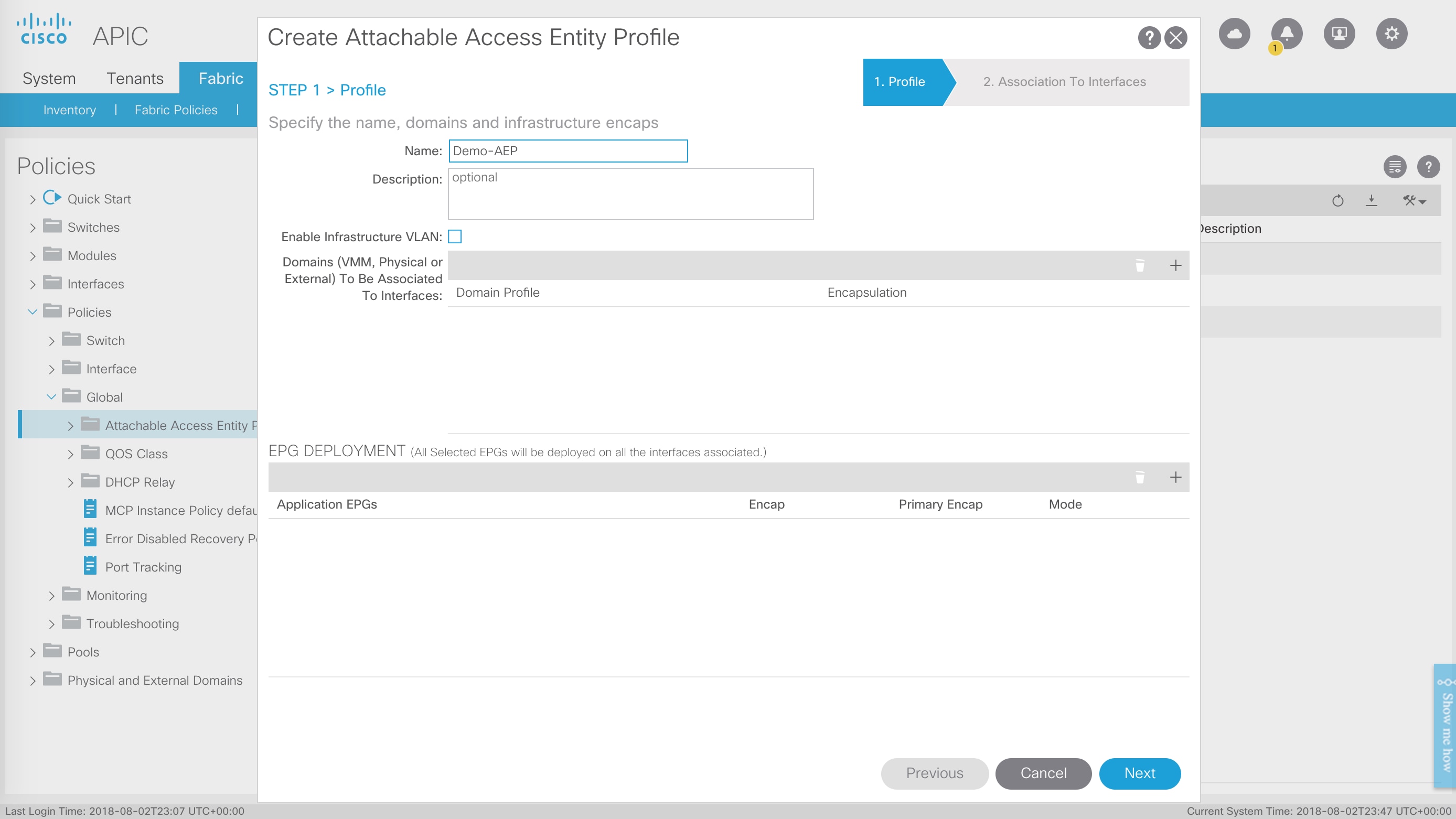This screenshot features a Cisco APIC (Application Policy Infrastructure Controller) interface with a prominent white pop-up menu at the center. The background of the website showcases a gray upper left corner with a blue icon made of dashes, followed by the blue text "Cisco" and the black text "APIC." 

Beneath the header, a vertical navigation menu is visible, listing options such as System, Tenants, and Fabric—with the Fabric section selected. Within the Fabric menu, items like Inventory, an unreadable option, Policies, Quick Start, Switches, Modules, Interfaces, Policies, Switch, Interfaces, Global, Attach Access Entity, Q05 Class, DHCP Relay, MCP Instance Proxy, Error, Disabled Recovery, Port Tracking, Monitoring, Troubleshooting, Pools, and Physical and External Domains are listed.

At the focal point of the screenshot, the white pop-up menu is titled "Create Attachable Access Entity Profile" in black font. Directly below the title, it reads "Step 1 Profile" in blue font, followed by instructions in black font to "Specify the Name, Domains, and Infrastructure."